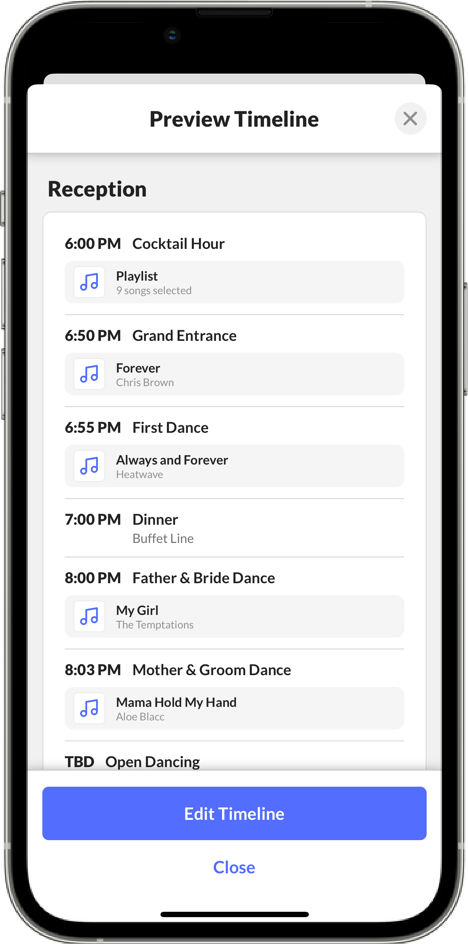The image captures a smartphone positioned screen-up, prominently displaying an event timeline on a white background. At the top is the title "Preview Timeline." Below, the schedule for a reception is meticulously detailed:

- 6:00 p.m.: Cocktail Hour with a playlist of nine selected songs.
- 6:50 p.m.: Grand Entrance featuring the song "Forever" by Chris Brown.
- 6:55 p.m.: First Dance to "Always and Forever" by Heat Wave.
- 7:00 p.m.: Dinner with a buffet line.
- 8:00 p.m.: Father and Bride Dance to "My Girl" by The Temptations.
- 8:03 p.m.: Mother and Groom Dance to "Mama Hold My Hand" by Aloe Blacc.
- TBD: Open Dancing.

A prominent blue rectangle with the text "Edit Timeline" in white spans across the screen, followed by the option "Close" in blue letters. The image, oriented taller than it is wide, contains no humans, animals, plants, buildings, vehicles, signs, or airplanes, emphasizing the digital focus.